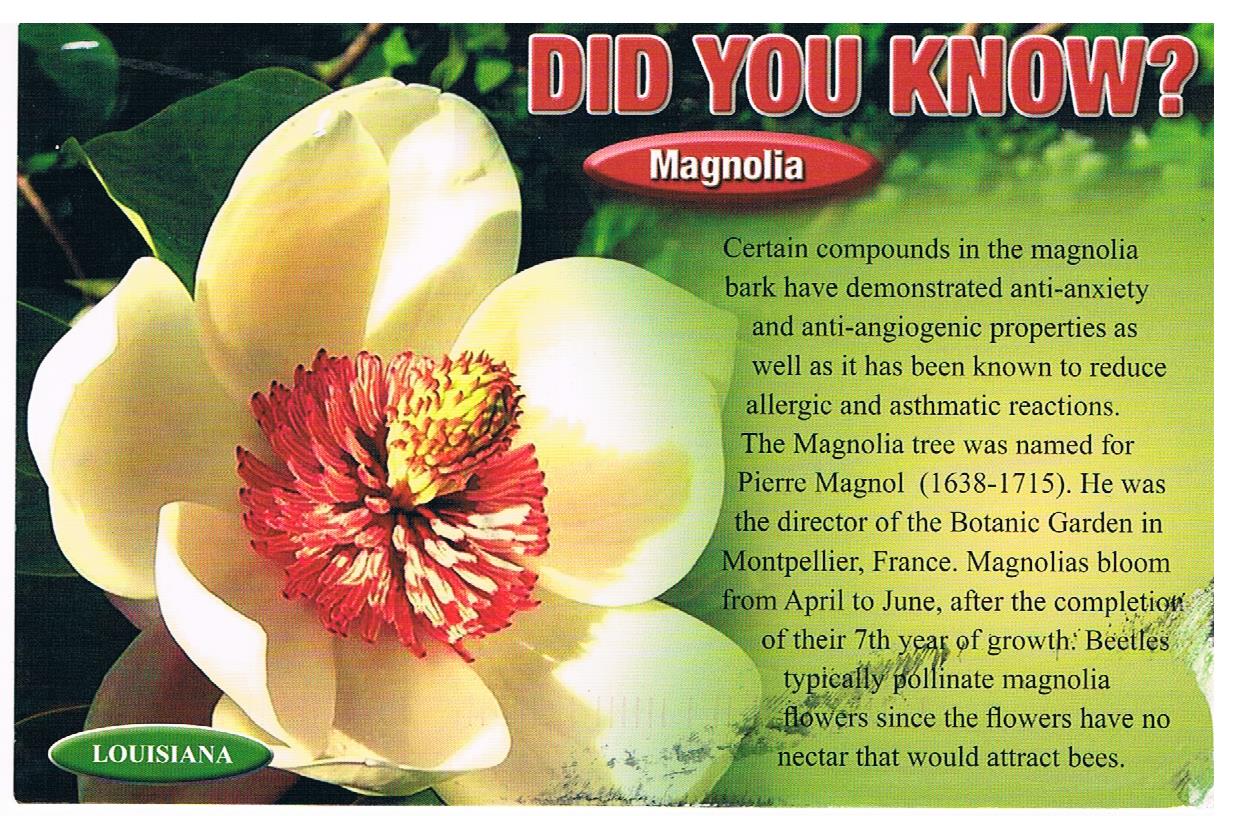This detailed infographic features an advertisement for the magnolia flower, with a bright, sunlit image of the flower dominating the left side. The magnolia in the photo is characterized by its pristine, round white petals encircling a red, petal-like core topped with a small, yellow-orange spiky section. Behind the flower, green leaves are visible, adding depth to the picture. 

On the top right corner of the image, the text "DID YOU KNOW" appears in all red, capital letters, followed by a smaller oval text box stating "Magnolias." The right side of the image has a green blurred background where informative text provides a wealth of details about the magnolia. It explains that compounds found in magnolia bark have been shown to have anti-anxiety and anti-angiogenic properties, and can also reduce allergic and asthmatic reactions. 

The magnolia tree is named after Pierre Magnol (1638-1715), who served as the director of the Botanic Garden in Montpellier, France. Additionally, it notes that magnolias typically bloom from April to June, reaching this stage after their seventh year of growth. It also mentions that beetles are the primary pollinators of magnolia flowers, as the flowers lack nectar to attract bees.

In the bottom left corner of the image, a green oval containing the word "LOUISIANA" in all capital white letters ties the advertisement to its regional context. Overall, the image and accompanying text serve to both inform and educate viewers about the distinctive features and benefits of the magnolia plant.